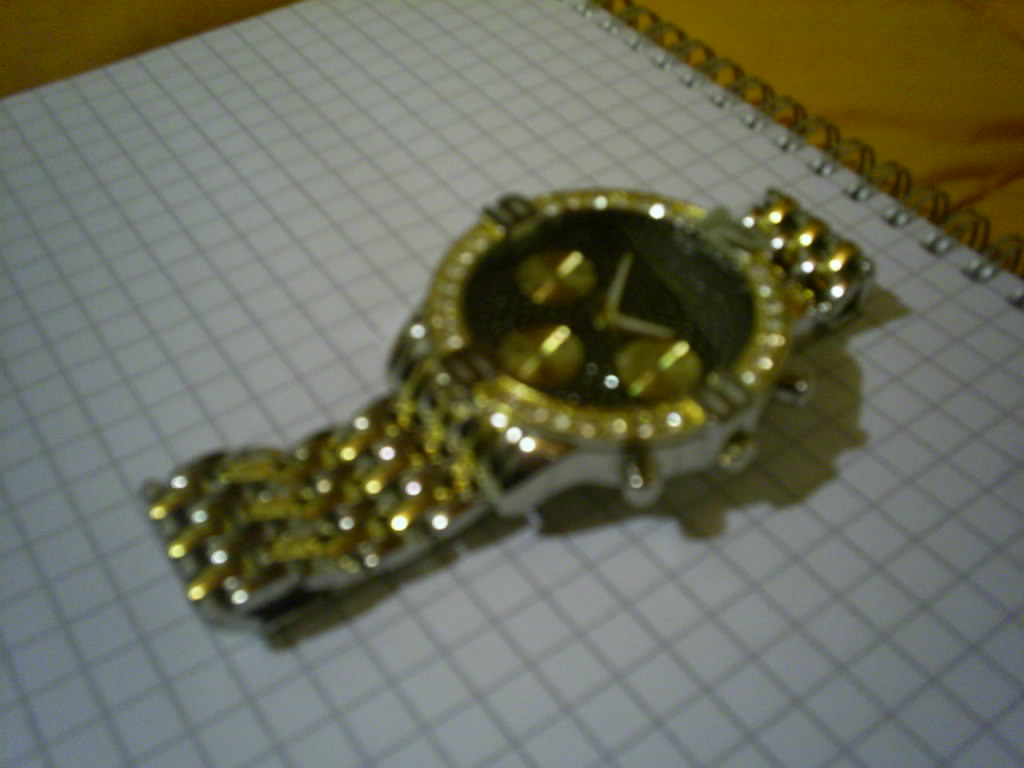This horizontal, rectangular color photograph, though slightly out of focus, features a detailed and ornate two-tone wristwatch. The watch, with an alternating gold and stainless steel band, is positioned diagonally across a spiral notebook filled with graph paper. The notebook lies on a tan wooden tabletop, with its spiral edge running from near the center of the top edge to almost the center of the right edge.

The main focal point, the watch, is shown prominently in the center, angled so that part of the band faces the upper right corner and part faces the lower left corner. Its black face is adorned with three smaller gold dials, and two gold hands indicate the time, which appears to be around 10 minutes before 2. The bezel of the watch is gold, complemented by three silver-looking buttons on its right-hand side. The watch's band, folded slightly underneath, showcases an interlinking pattern of gold and stainless steel.

A shadow cast by the watch is visible to its right, enhancing the image's depth. The blurred edges of the photograph reveal snippets of the tan wooden tabletop in the upper right and left corners. Despite the slight blur, the photograph captures the intricate details of the watch and the utilitarian, yet neatly arranged setup of the graph paper notebook on which it rests.